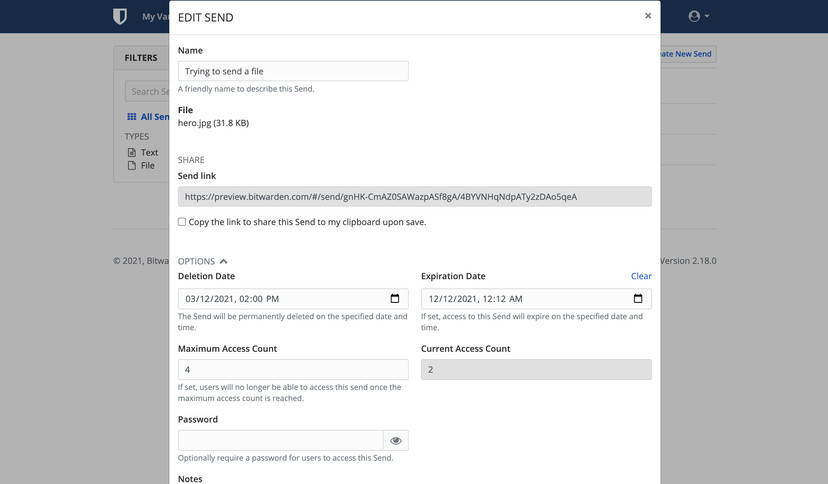This is a detailed screenshot of a web interface, possibly from a file sharing or management platform. The central focus is a large white overlay window titled "Edit Send." The window appears to be managing the settings for sharing a file. 

The window displays the following fields and details:

- **Name:** Indicates the user is in the process of sending a file.
- **Description:** A friendly name to describe this send.
- **File:** A .jpg file with a size of 31.8 KB.
- **Share:** Includes a link for sharing: `https://preview.bitwarden.com`, repeated multiple times.
- **Link Sharing Option:** Provides an option to copy the link to the clipboard upon save.
- **Options:**
  - **Deletion Date:** Specifies that the send will be permanently deleted on March 12, 2021, at 2 PM.
  - **Maximum Access Count:** Limits access to the send to a maximum of 4 times. Once reached, users can no longer access the file.
  - **Password:** Allows optionally requiring a password for users to access the send.
  - **Notes:** May include additional details.
  - **Expiration Date:** Sets an expiration for the send on December 12, 2021, at 12:12 AM.
  - **Current Access Count:** Indicates the file has been accessed 2 times so far.

The underlying website remains unidentified due to the overlay obscuring the background content.